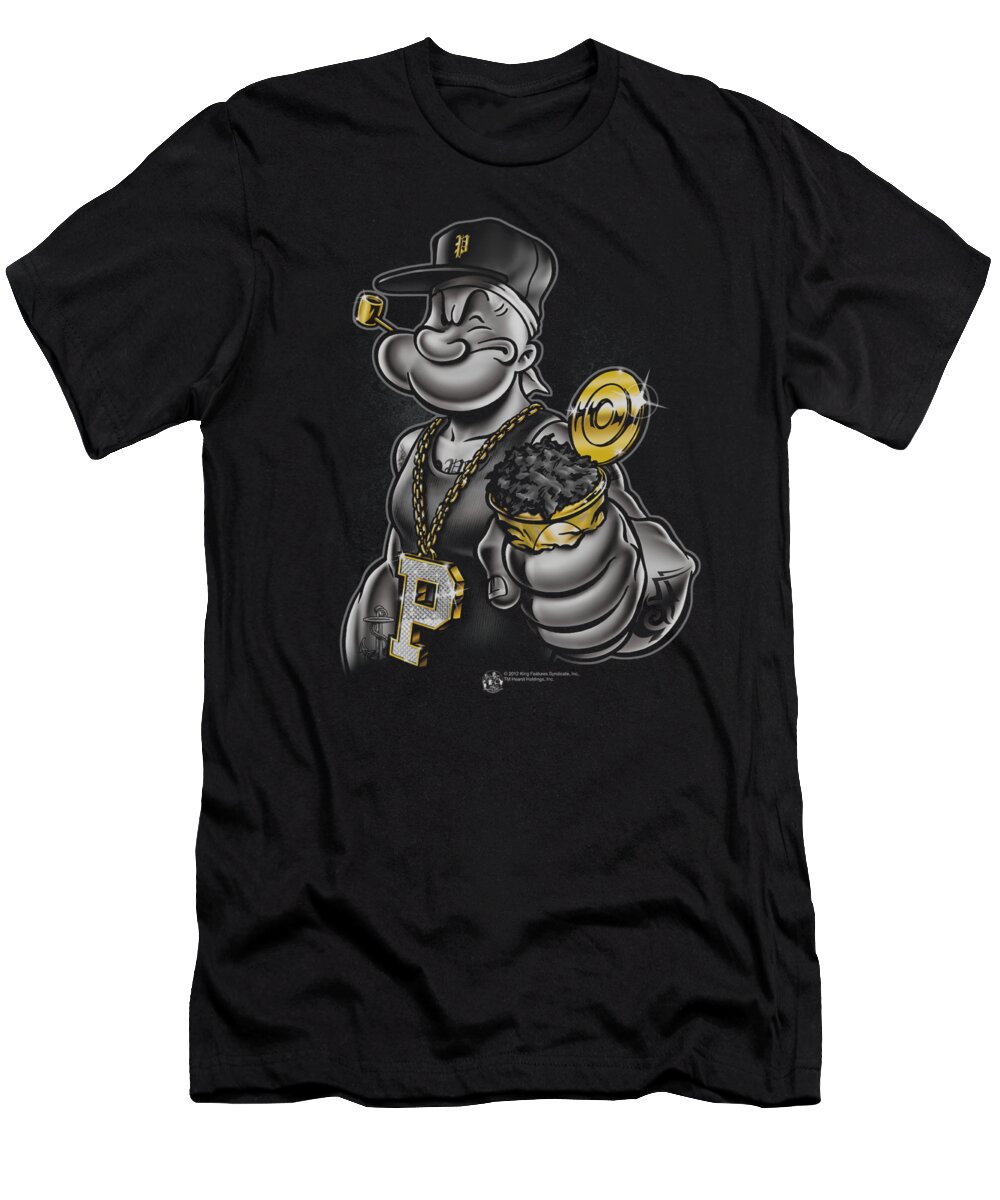The image features a men's crew neck t-shirt in solid black, laid flat against a pure white background. The shirt is slightly wrinkled and tagless. The chest area boasts a detailed printed design of the classic cartoon character Popeye. Rendered primarily in black and white, Popeye is depicted with his characteristic squinting eyes and a broad smile. He wears a black baseball cap embellished with a gold logo featuring the letter "P," possibly representing the Pittsburgh Pirates. A gold chain with a large capital "P" as the pendant hangs around his neck, matching the gold highlights on his hat. Popeye holds a golden tin can in his left hand, from which black spinach protrudes. Completing the design, a gold pipe extends from the right side of his mouth. There may be some barely discernible trademark text beneath the image.